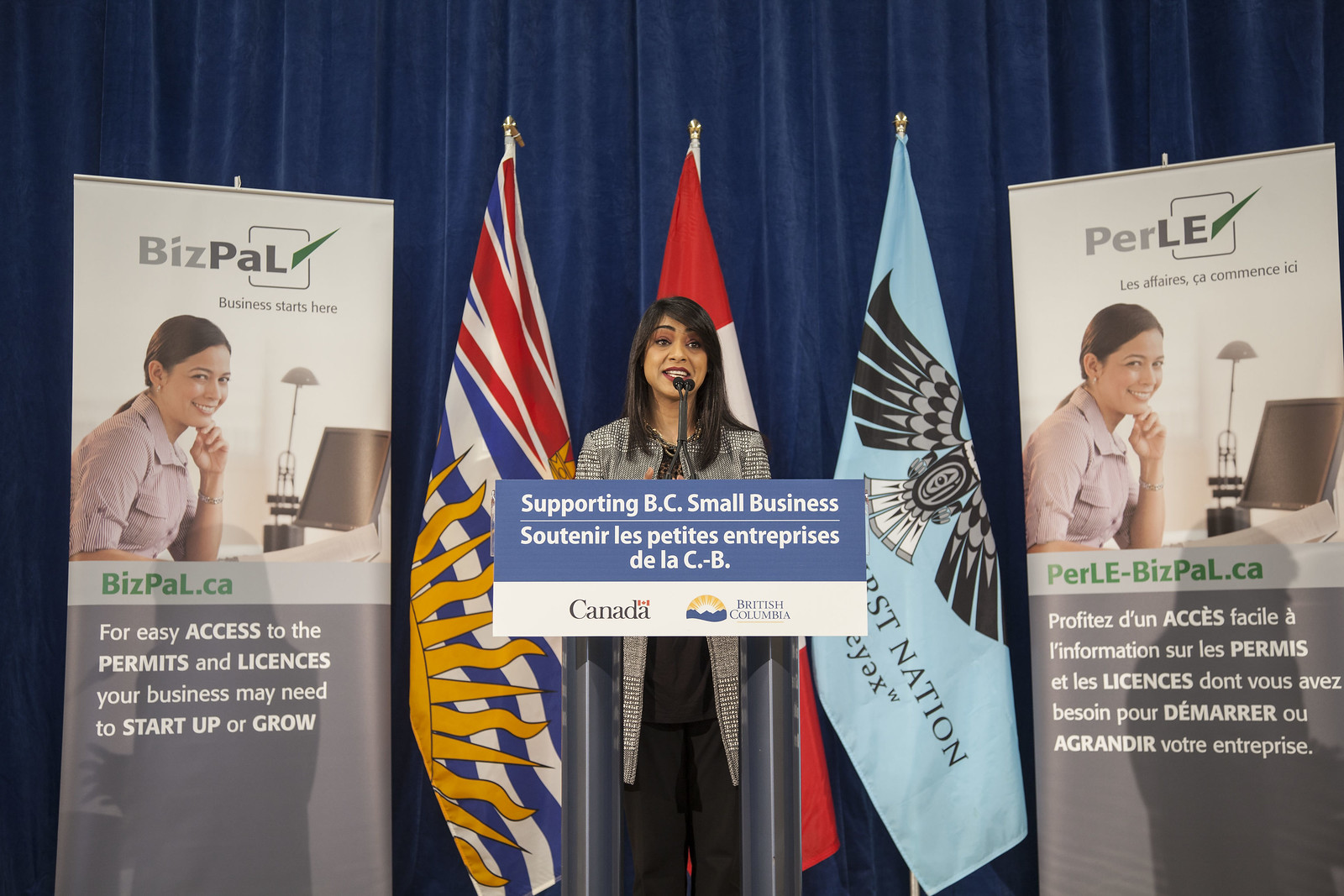The image depicts a detailed scene of a press conference where a woman is speaking at a podium, which conveys a robust support for small businesses in British Columbia. The podium, comprised of two gray posts supporting a large blue and white sign, prominently reads "Supporting BC Small Business" with a French translation beneath it. Below these messages are the logos of Canada and British Columbia. 

The woman appears to be of Middle Eastern, Indian, or Latin descent, with brown skin and long, black hair parted to the side, flowing down to her shoulders. She is adorned with red lipstick, a black and white striped coat, a black shirt, and black pants. Her mouth is open as if she is caught mid-sentence, speaking from behind a microphone.

Behind her is a backdrop of a blue curtain, with three flags standing: the British Columbian flag on the left, the partially visible Canadian flag behind her, and a blue flag with an eagle and black writing to the right. Flanking her, beyond the flags, are large, upright posters that feature a woman smiling at a computer screen. These banners bear the "BizPal" logo, which promotes easy access to permits and licenses necessary for business startups and growth. The English version of the sign is on the left, and the French version is on the right, illustrating the bilingual nature of the event.